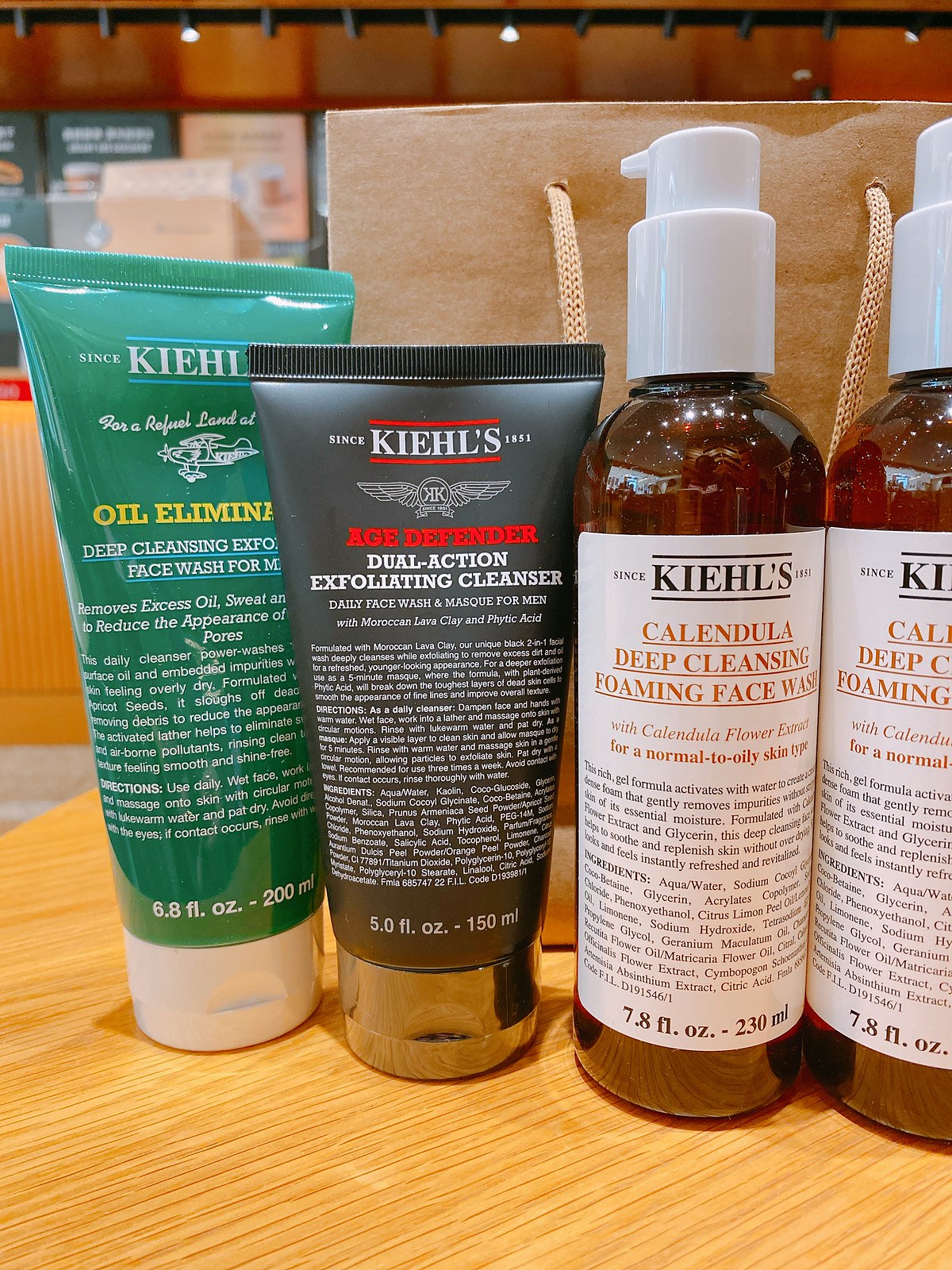A close-up image captures the back of various liquid skincare products arranged on a wooden tabletop. In the foreground, a brown paper shopping bag with cotton handles suggests a recent purchase. The background reveals a serving area and signage, indicating a mall eatery setting. 

Four products are displayed prominently:
1. On the right, two 230ml black circular cylinder bottles by Kiehl’s feature white push-pump lids and white back labels. The labels identify these as "Deep Cleansing Foaming Face Wash."
2. On the left, two green squeezy bottles also from Kiehl’s are present. The far-left light green bottle (200ml) is labeled "Oil Eliminating Deep Cleansing Exfoliate." Adjacent to it, the darker green bottle (150ml) is marked "Age Defender Dual-Action Exfoliating Cleanser."

Each product indicates its purpose as a face wash or cleanser, providing a peek into an assortment of Kiehl's skincare essentials for maintaining a clean and refreshed complexion.